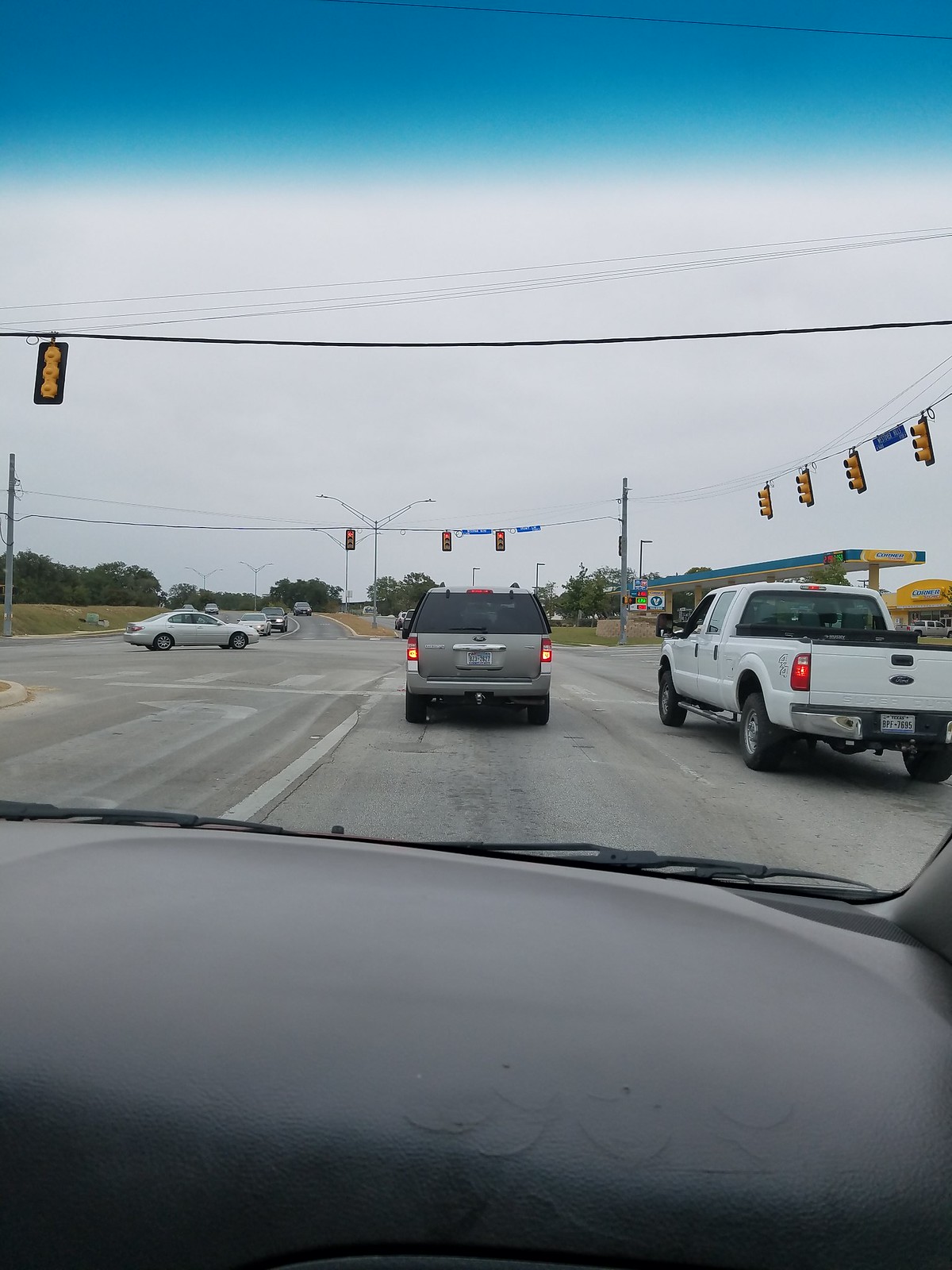The photograph captures the view from inside a vehicle, looking through the front windshield. The gray dashboard is prominently visible in the foreground, along with the windshield wipers lying flush against the glass. The road ahead is paved with gray asphalt, crowded with vehicles halted at a red light. Directly in front is a gray SUV, its brake lights aglow. To its right, a white extended cab truck also waits, its brake lights similarly illuminated. The traffic lights that have brought the procession to a halt can be seen suspended from wires above the intersection.